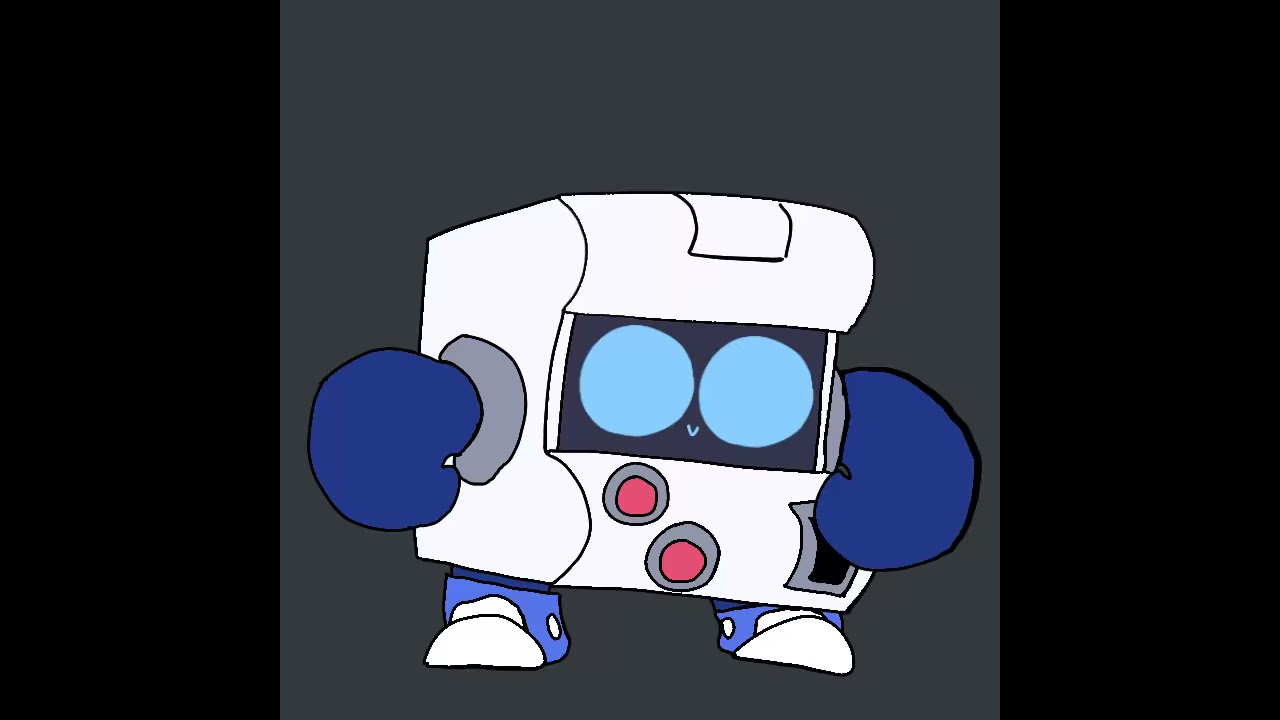The image is a cartoonish, computer-drawn graphic of a small robot that resembles a game or vending machine. This white-bodied robot, shaped somewhat like a square toaster, features a black screen inset in its body. It has two large, light blue circular eyes and a tiny V-shaped mouth positioned between them, creating a simple, friendly expression. Below the eyes on the white part of the body are two red buttons bordered by gray rings, possibly resembling a coin slot.

The robot's hands are depicted as blue boxing gloves, suggesting a playful or fighting theme, while its feet are blue and white sneakers. The entire robot is set against a dark charcoal gray background, and black rectangles flank its sides. The overall appearance is reminiscent of an arcade character, ready for action.